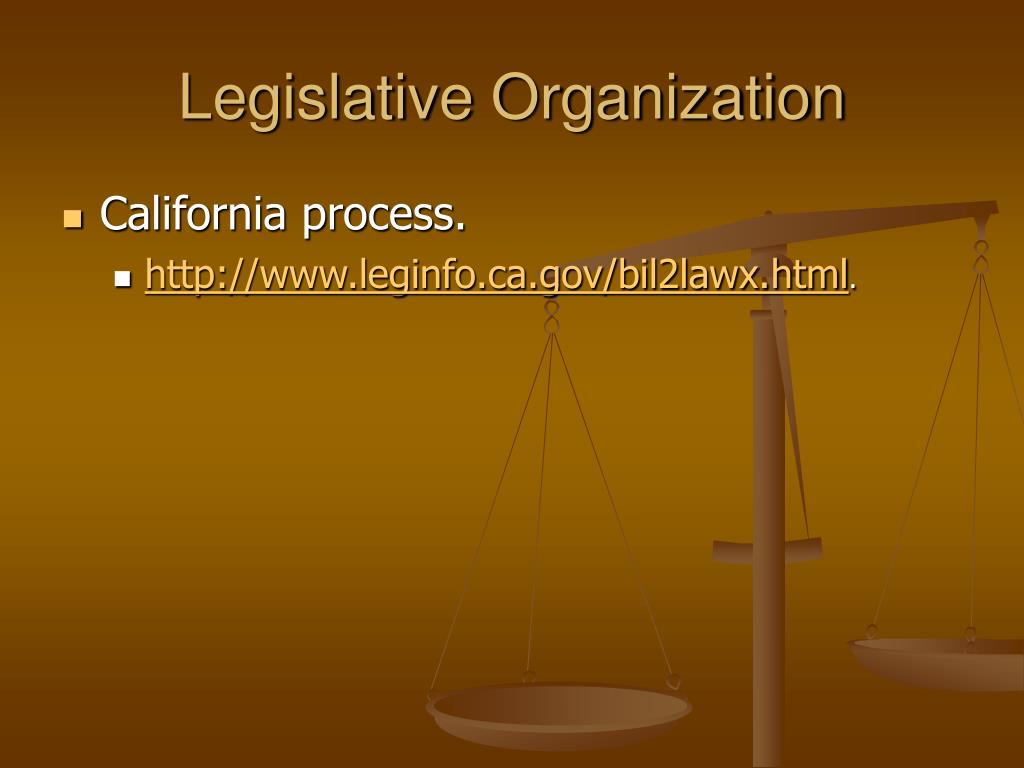The image depicted is a detailed capture from a PowerPoint slide that focuses primarily on textual information. The background features a gradient of brown shades, starting with a regular brown at the edges, lightening at the center, and darkening again towards the bottom, creating a tannish effect. In the bottom-right corner, there is an illustration of an old-school balance scale depicted in a dark beige color, complete with a central cylinder, a crossbar, hooks, chains, and dual bowls. The slide carries the heading "Legislative Organization" in either light brown or blue font, located prominently at the top. Below this, in white font, is a subheading "California Process," followed by the website URL "http://www.leginfo.ca.gov/bil2lawx.html." The setting of the slide indeed suggests it is part of an informative presentation. The colors in the image predominantly include various shades of brown, tan, beige, and white.